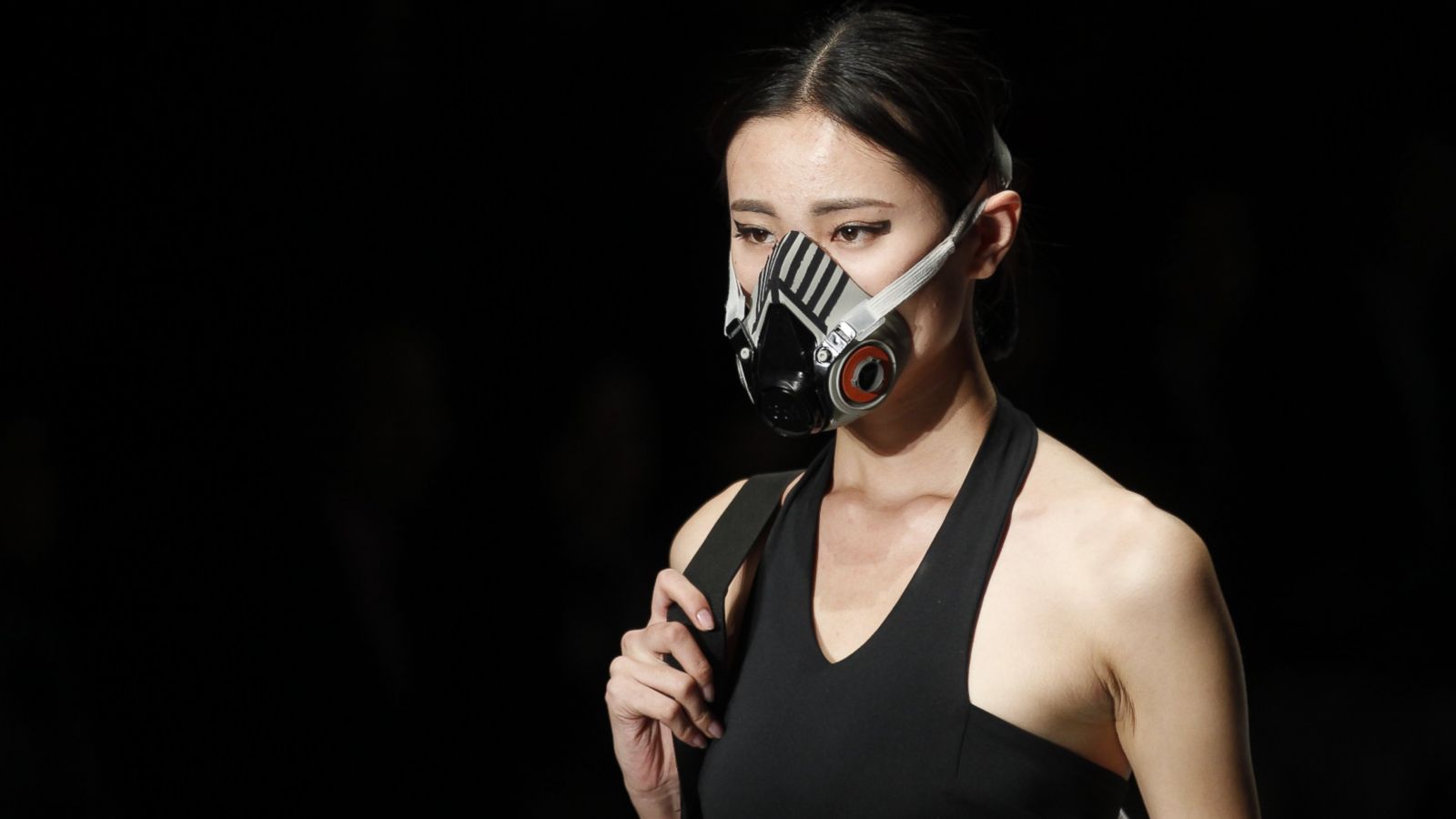This image captures a striking portrayal of an Asian woman against a completely black background, emphasizing her as the focal point with no visible distractions behind her. The woman is lit quite dramatically, suggesting she might be a runway model or participating in a photo shoot. She is depicted from the chest up, wearing a thin-strapped black top. Her hair is neatly pulled back into a bun, while her eyes are heavily accentuated with extensive eye makeup, highlighting her striking gaze.

The most prominent feature of the photograph is the elaborate mask covering her mouth and nose. This mask appears to be a sophisticated, rubberized, black, white, and brown contraption, potentially a breathing regulator, complete with replaceable filters and a red circular aperture on the side for attachments. The mask is secured with thick, predominant white straps that extend around the back of her head, attached via metal swivels to a plastic clip and then to an elastic band ensuring a firm fit. In her raised right hand, near her shoulder, she holds another strap, possibly from a bag or an accessory, natural-colored nails visible. The overall composition, lighting from the left and front, and the intricate details of her mask create a profound and visually captivating image.